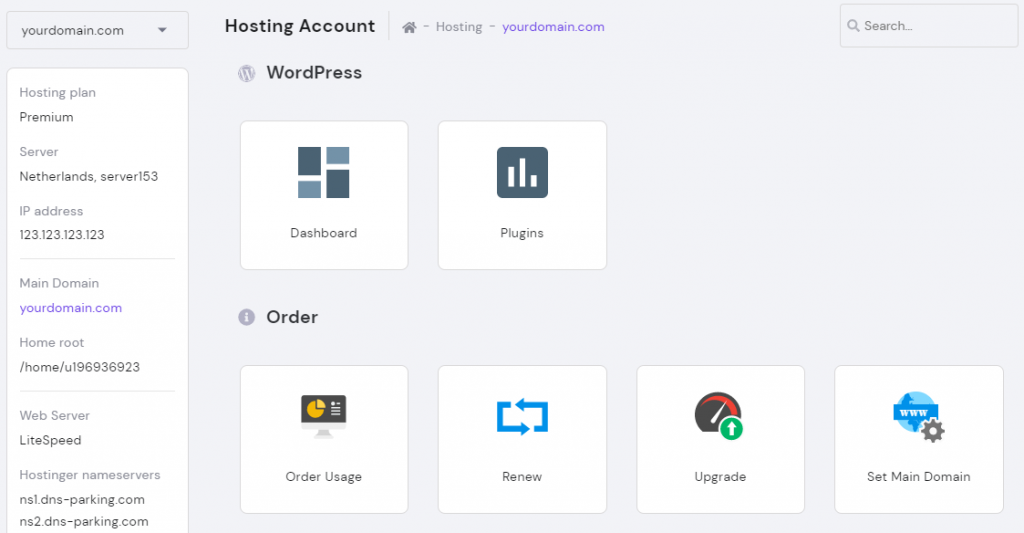This screenshot captures a web page with a light gray background. In the upper left corner, there is a gray rectangle containing the text "yourdomain.com" in gray font. To the right of this, an arrow points downwards, indicating a drop-down menu. Moving further right, the phrase "Hosting Account" is displayed in black font. Below this, a horizontal gray line is followed by a small gray house icon. Adjacent to the icon, separated by dashes, the word "Hosting" is printed, and another dash leads to "yourdomain.com" in blue font. 

In the upper right corner, there is a subtle search field, matching the background color. It contains the placeholder text "Search..." in gray font, accompanied by a gray magnifying glass icon to its left.

The main content area of the page has several white squares arranged on the light gray background. The first row is labeled "WordPress," containing two squares: one labeled "Dashboard" with an icon of four small gray squares, and the other labeled "Plugins," featuring a dark gray square with a white bar graph icon. Below this row is another section labeled "Order."